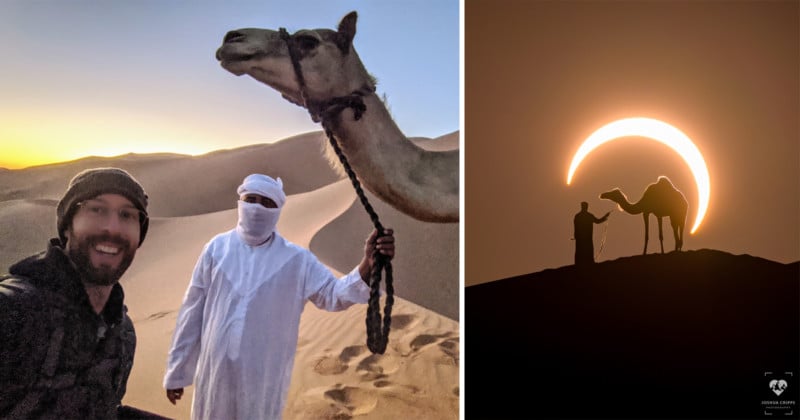In this landscape-oriented collage, two photographs are divided by a vertical white line. On the left, a bearded man wearing glasses, a brown beanie, and a dark jacket stands in the corner of the frame, capturing a selfie. Beside him is a figure dressed in traditional white Bedouin attire, with only his eyes visible through his headdress and mask. This figure holds a rope attached to a camel whose head appears just above him. The background reveals a stretch of uninterrupted sand dunes under a blue sky tinged by the setting sun. The right photograph presents a striking silhouette scene, featuring the same man and camel against the backdrop of an eclipse. The landscape below is in shadow, with the darkened land forming a silhouette. Above, the solar eclipse partially obscures the sun, creating a crescent of light in an orangey-brown sky. The carefully staged composition highlights the dramatic contrast between the serene desert day and the eerie, shadowy eclipse.